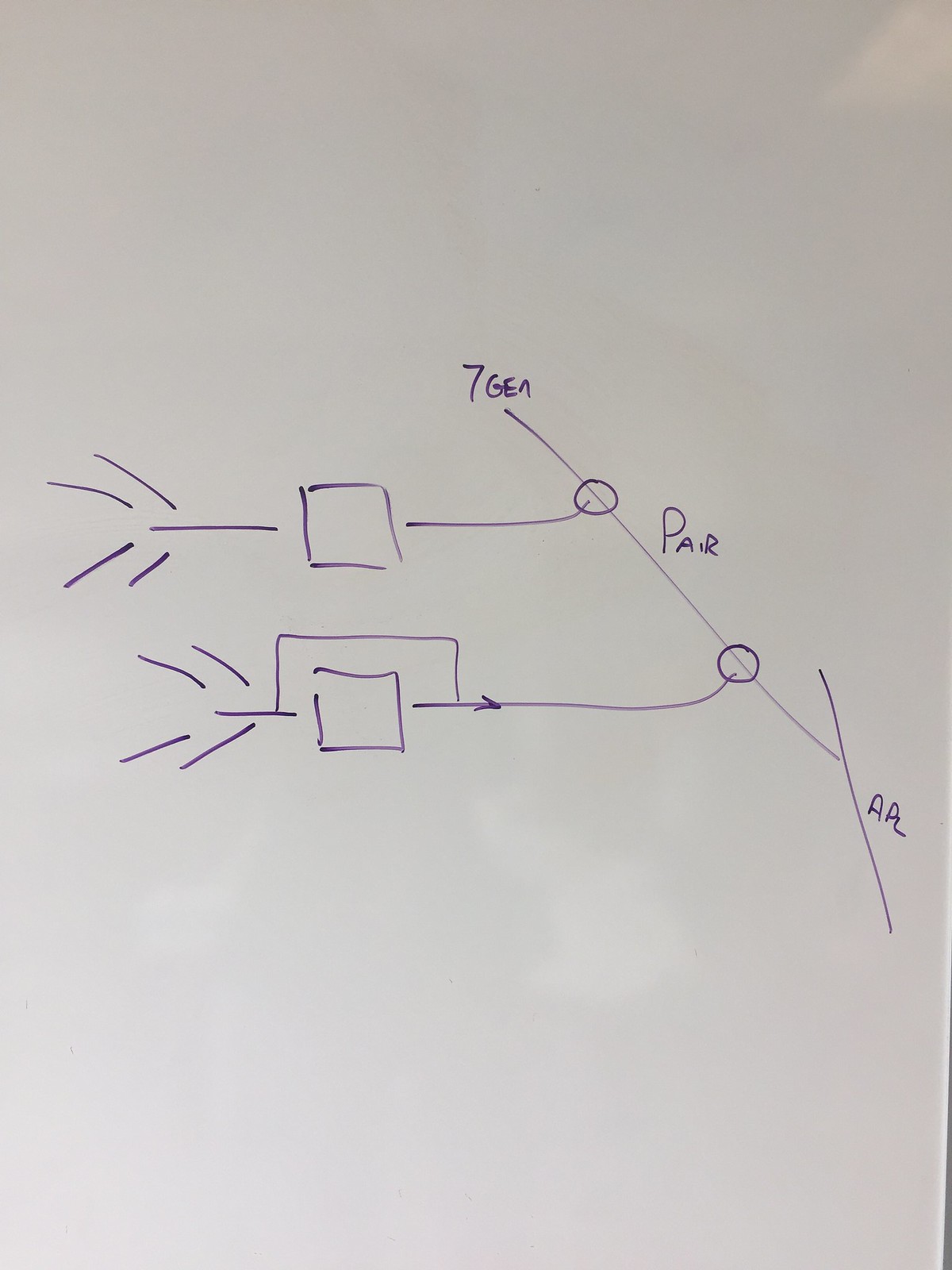The image displays what appears to be a standard 8.5x11 inch piece of printer paper, although it could also be a whiteboard due to the nature of the markings. The background is white but not exceptionally bright. It is adorned with handwritten notes in a medium to dark, yet fairly bright, purple color, likely made with a dry erase marker.

At the top of the image, the text "7gen" is written, potentially signifying "seventh generation." Below this, a slanting line descends diagonally, labeled "pair" at a midpoint. At the bottom end of this line, another horizontal slash is marked with "AP2" or possibly "APL."

Beneath the horizontal slash, there is a small circle connected by a line to a square, both drawn in the same purple marker. To the left of the square, several purple lines resembling the fletching of an arrow fan outwards. 

A similar diagram is replicated lower down, diagonally to the left beneath the word "pair." This secondary image features a square with a partially obscured rectangle behind it, situated along the slanting line. There also appears to be a small arrow pointing towards a circle.

The handwriting throughout is not particularly clear, but the symbols and structure suggest the depiction of a mathematical, genetic, or scientific formula.